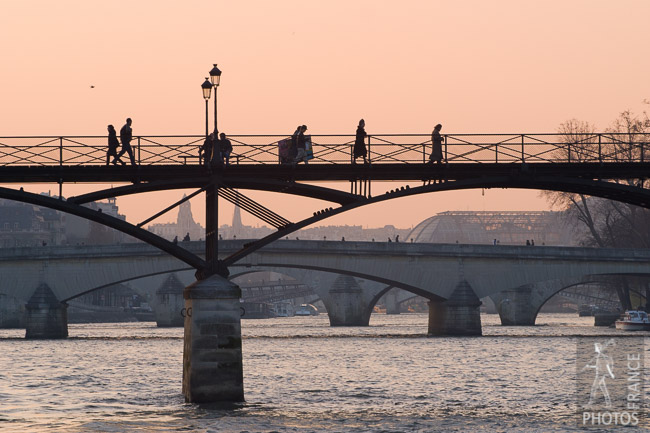This photograph, likely taken in France as suggested by the "photos France" watermark in the bottom right corner, features a serene scene at dusk. The orange-pink sky casts a warm, ethereal light over the setting. In the foreground, there's an iron pedestrian bridge with metal railings and arches, supported by a massive stone pillar. The bridge is adorned with two black metal light posts and you can see the silhouettes of several people walking across it, as well as two individuals seated on a bench. Below, blue rippling water flows gently under the bridge. Further in the background, there are several more bridges—one of which is a larger, concrete bridge potentially accommodating both pedestrians and vehicles. Tiny figures can be seen walking across this larger bridge, emphasizing its scale. Beyond these layers of bridges, the faint silhouettes of cone-shaped towers and distant buildings loom, adding depth to the sprawling cityscape. Additionally, a couple of boats are visible on the water, enhancing the picturesque urban river setting.